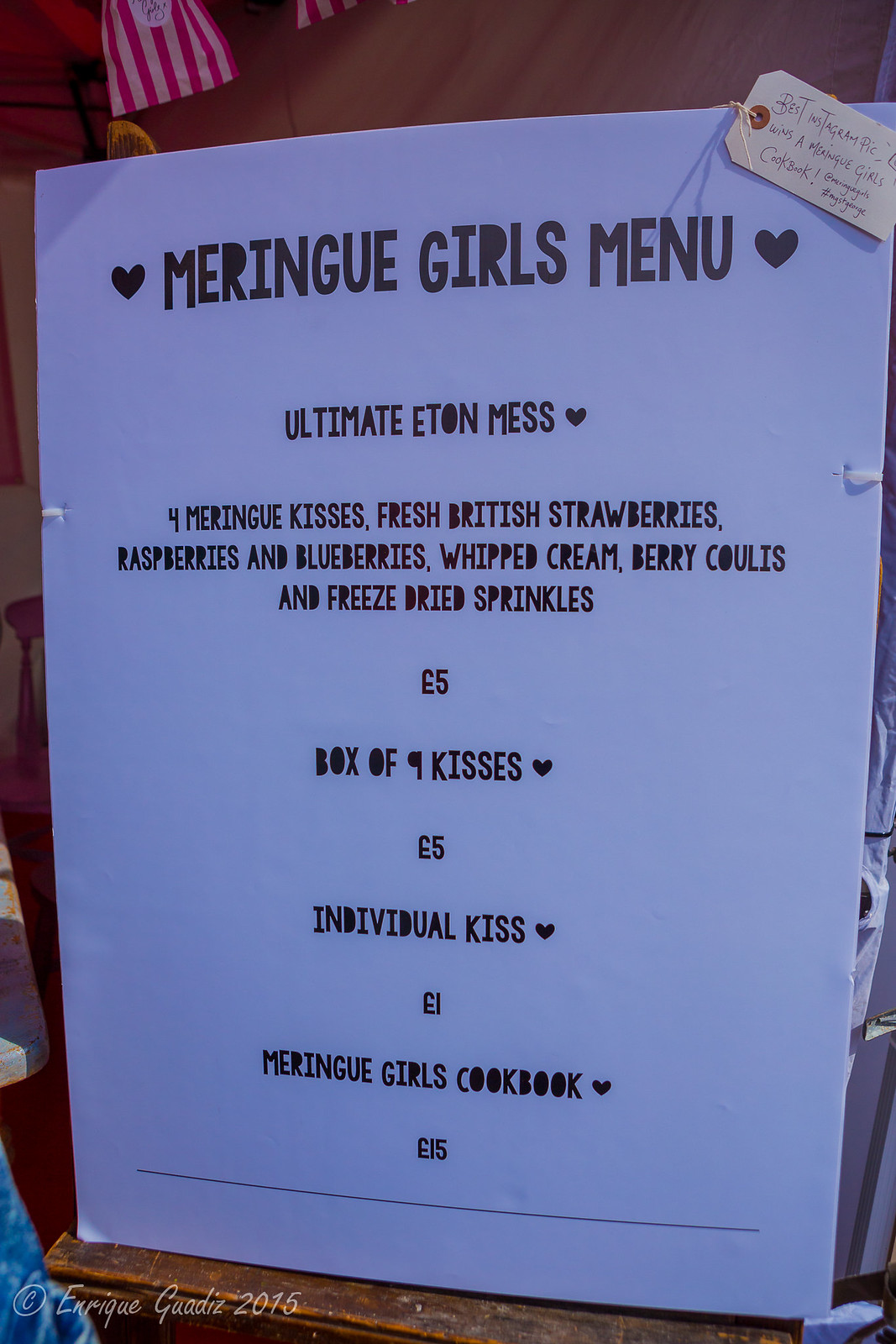The photograph showcases a piece of white paper with black ink, displayed on what seems to be a wooden shelf. The top of the paper features two small hearts flanking the title "Meringue Girls Menu." Beneath the title, the menu advertises the "Ultimate Eton Mess," which includes four Meringue Kisses, fresh British strawberries, raspberries, and blueberries, whipped cream, berry coulis, and freeze-dried sprinkles, priced at five pounds. Additional items on the menu include a box of nine Meringue Kisses for five pounds, an individual Meringue Kiss for one pound, and the "Meringue Girls Cookbook" for fifteen pounds. Below this, a note indicates a promotional tag reading “Best Instagram Pick Wins a Meringue Girls Cookbook,” with a prompt to tag @MeringueGirls and hashtag #MGSTGeorge. The bottom left corner of the paper is marked with “Copyright Enrique Gardi, 2015,” presumably crediting the photographer. The scene also includes glimpses of a white and pink striped cloth and bits of a tagged note in the background.